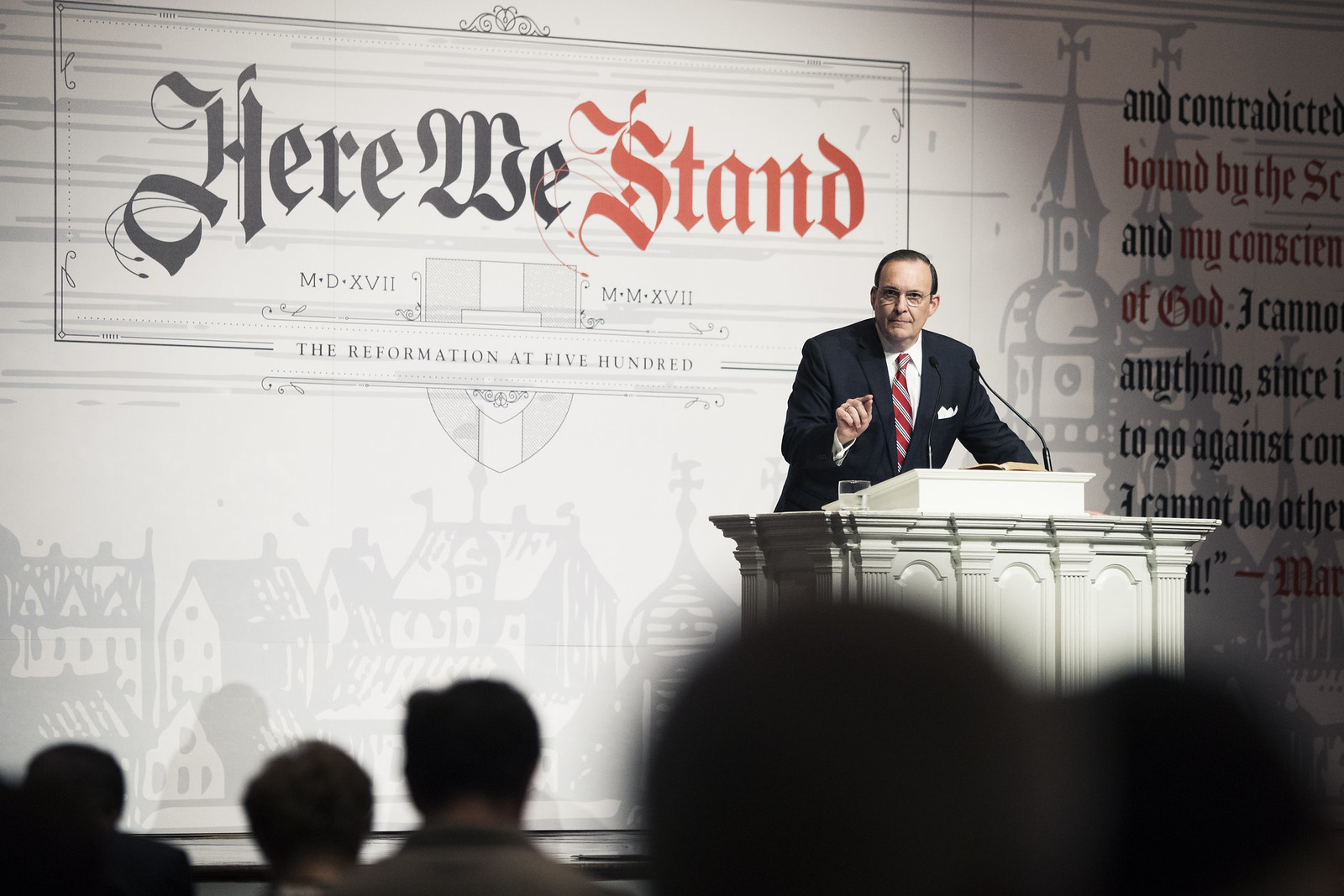The photograph captures a man in a black suit, white dress shirt, and silver and red striped tie, standing behind a religiously designed white podium at what appears to be a church-like setting. He is wearing glasses and pointing two fingers towards the crowd, with a microphone and a glass of water on the podium. The darkened silhouettes of the audience heads are visible in the foreground. Behind the speaker is a backdrop featuring the bold words "Here We Stand" with "stand" emphasized in red, and the symbols "MDXVII, MMXVII. The Reformation at 500." Additionally, the background displays intricate graphics of cathedral domes, turrets, crosses, and steeples. Partially visible text reads, "and contradicted, bound by the... and my conscience of God... anything since... to go against... cannot do other." The bottom corner appears to reference a religious text, possibly starting with "Mark" or "Matthew."